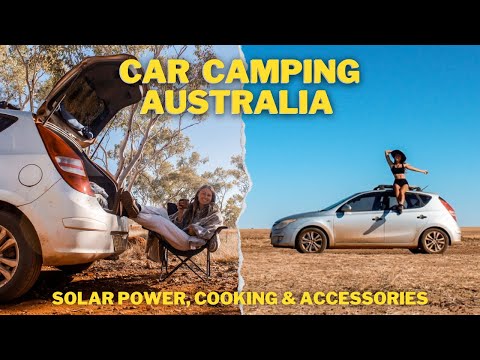The promotional image, framed by thin black bars at the top and bottom, features large yellow text reading "Car Camping Australia." Below that, in smaller yellow print, are the words "Solar Power, Cooking, and Accessories." The image consists of two panels. The left panel shows the rear of a small silver four-door compact car with the hatch open, where a Caucasian woman, dressed in a sweatshirt and long pants, is smiling and enjoying a beverage while seated on a lounge chair amidst a backdrop of trees. Her feet are propped against the car. The right panel depicts a second photo of the same woman, now in a different setting under a bright blue sky. She is sitting on top of the car, wearing a two-piece bathing suit, a black sun hat, and black shoes, showcasing her midriff. This scene appears to be in a more open, possibly desert-like area. The image collectively illustrates the contrast and versatility of car camping in Australia, highlighting solar power, cooking, and various camping accessories.